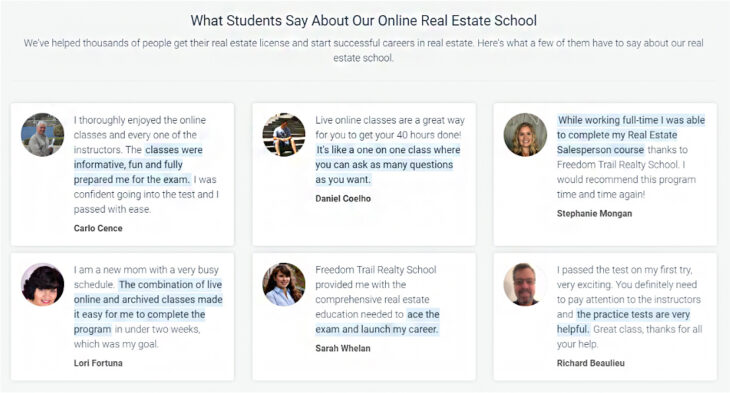Screenshot of an Online Real Estate School Testimonials Page

This image captures a screenshot from an unidentified website featuring testimonials for an online real estate school. The header at the top reads, "What Students Say About Our Online Real Estate School." A brief description follows, stating that the school has helped thousands obtain their real estate licenses and embark on successful careers. It invites readers to explore the experiences of a few students.

The main section of the page, set against a grayish-white background, displays six student testimonials. Each testimonial is presented in a white box and accompanied by a circular photo of the student and their name highlighted below their testimonial. Key phrases within the testimonials are emphasized using light blue highlight and bold text to make them stand out.

### Detailed Breakdown of Testimonials:

- **Top Left: Carlo Cent**
  - **Testimonial:** "I thoroughly enjoyed the online classes and every one of the instructors. The classes were informative, fun, and fully prepared me for the exam. I was confident going into the test and I passed with ease."
  - **Highlighted:** "classes were informative, fun, and fully prepared me for the exam."

- **Top Middle: Daniel Colho**
  - **Testimonial:** "Live online classes are a great way for you to get your 40 hours done. It's like a one-on-one class where you can ask as many questions as you want."
  - **Highlighted:** "it's like a one-on-one class where you can ask as many questions as you want."

- **Top Right: Stephanie Mongan**
  - **Testimonial:** "While working full-time, I was able to complete my real estate salesperson course thanks to Freedom Trail Realty School. I would recommend this program time and time again."
  - **Highlighted:** "while working full-time, I was able to complete my real estate salesperson course thanks to Freedom Trail Realty School."

- **Bottom Right: Richard Beaulieu**
  - **Testimonial:** "I passed the test on my first try. Very exciting. You definitely need to pay attention to the instructors. The practice tests are very helpful. Great class, thanks for all your help."
  - **Highlighted:** "the practice tests are very helpful."

- **Bottom Middle: Sarah Whelan**
  - **Testimonial:** "Freedom Trail Realty School provided me with the comprehensive real estate education needed to ace the exam and launch my career."
  - **Highlighted:** "ace the exam and launch my career."

- **Bottom Left: Lori Fortuna**
  - **Testimonial:** "I am a new mom with a very busy schedule. The combination of live online and archived classes made it easy for me to complete the program in under two weeks, which was my goal."
  - **Highlighted:** "the combination of live online and archived classes made it easy for me to complete the program."

This well-organized layout, featuring highlighted key points and personal photos, allows prospective students to easily grasp the value and effectiveness of the online real estate courses offered by this school.